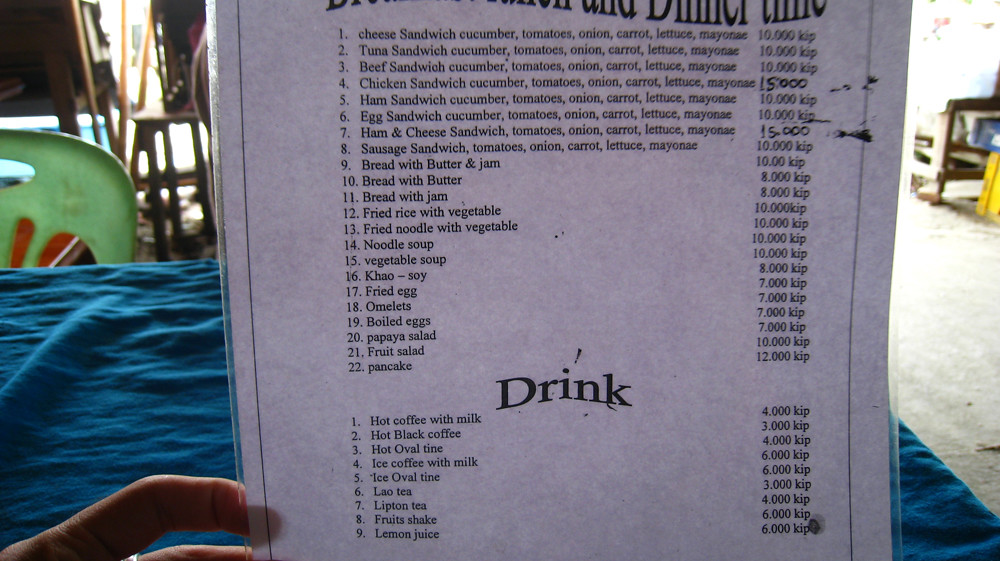This is a vivid color photograph capturing a close-up view of a portion of a menu held by a person with very pale skin. Only the thumb and index finger of this individual are visible, firmly grasping the slate gray menu on the left side. The menu itself is printed in delicate black text. The backdrop reveals a glimpse of a table adorned with an elegant turquoise blue tablecloth, adding a pop of color to the scene.

The detailed menu lists various food and drink items. The food section starts with "Bread with Butter," followed by options such as "Bread with Butter and Jam," "Sausage Sandwich," "Tomatoes, Onion, Carrot, Lettuce, Mayonnaise," "Fried Noodles with Vegetables," "Noodle Soup," "Vegetable Soup," "Omelet," "Boiled Eggs," "Papaya Salad," "Fruit Salad," and "Pancake." Below the food items, a headline reads "Drink," under which choices like "Hot Coffee with Milk," "Hot Black Coffee," "Hot Ovaltine," "Iced Ovaltine," "Lemon Juice," and "Protein Shake" are listed.

The photograph highlights the juxtaposition of the gray menu and the turquoise tablecloth, emphasizing the tactile interaction between the diner and the menu, as well as providing an enticing glimpse into the varied offerings of the establishment.